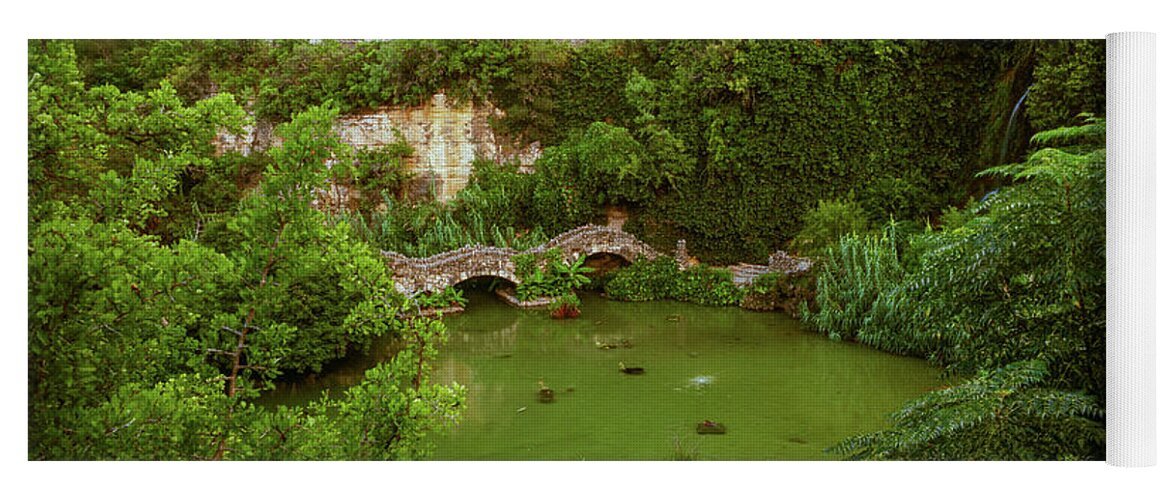A distant, aerial photo captures a lush, ancient scene dominated by a verdant green landscape. Central to the image is a wavy, stone footpath bridge with an arched design, composed of interconnected stones. The bridge spans a shallow, slow-moving river, tinged green likely due to algae or pollen. This river contains several small islands or rocks, adding to the picturesque nature of the scene.

Surrounding the bridge, on both sides, is dense, jungle-like vegetation with an array of dark green, healthy trees and thick plant growth. Behind the bridge rises a white, bleached cliff, partially obscured by rich, green foliage. Atop and around this cliff is abundant plant life contributing to the overall verdant ambiance. 

The background features a beige stone wall, adding a sense of antiquity. This combination of natural and ancient man-made elements evokes a setting that appears to be from a distant land, possibly resembling landscapes found in Asia. Rocks and greenery in the foreground frame this serene, timeless scene.